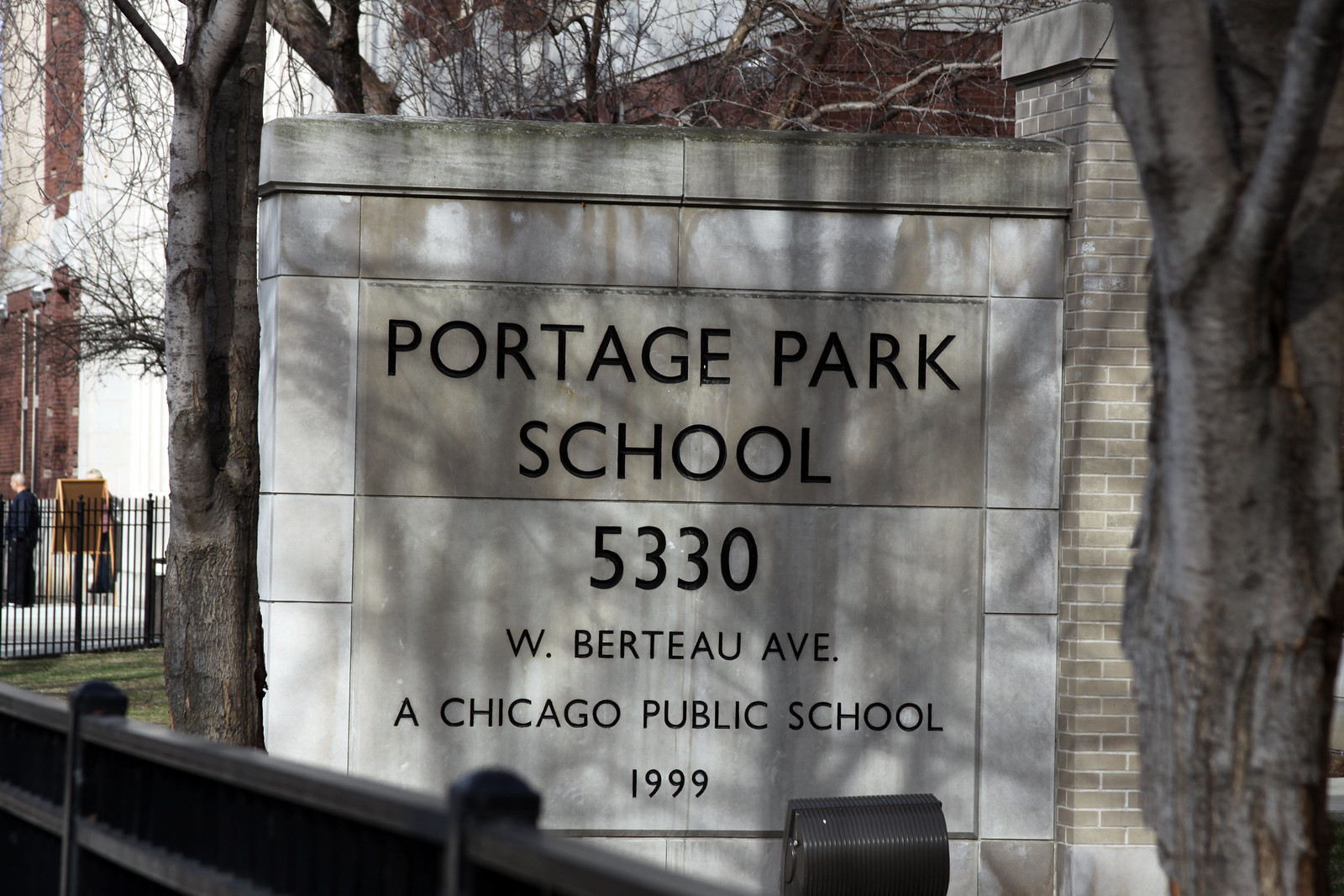The image captures an outdoor scene featuring a cement sign with engraved, black lettering that reads "Portage Park School, 5330 West Berteau Avenue, a Chicago Public School, 1999." The sign, which is off-white, stands prominently in the center of the image. Flanking the sign, there are trees on both sides, with a particularly large tree being on the right side in the foreground. In the background, the top of a brick building is visible. The area in front of the sign is enclosed by a black metal guardrail. Additionally, to the left of the sign, a person dressed in black can be seen in the distance, behind another section of the metal fence.